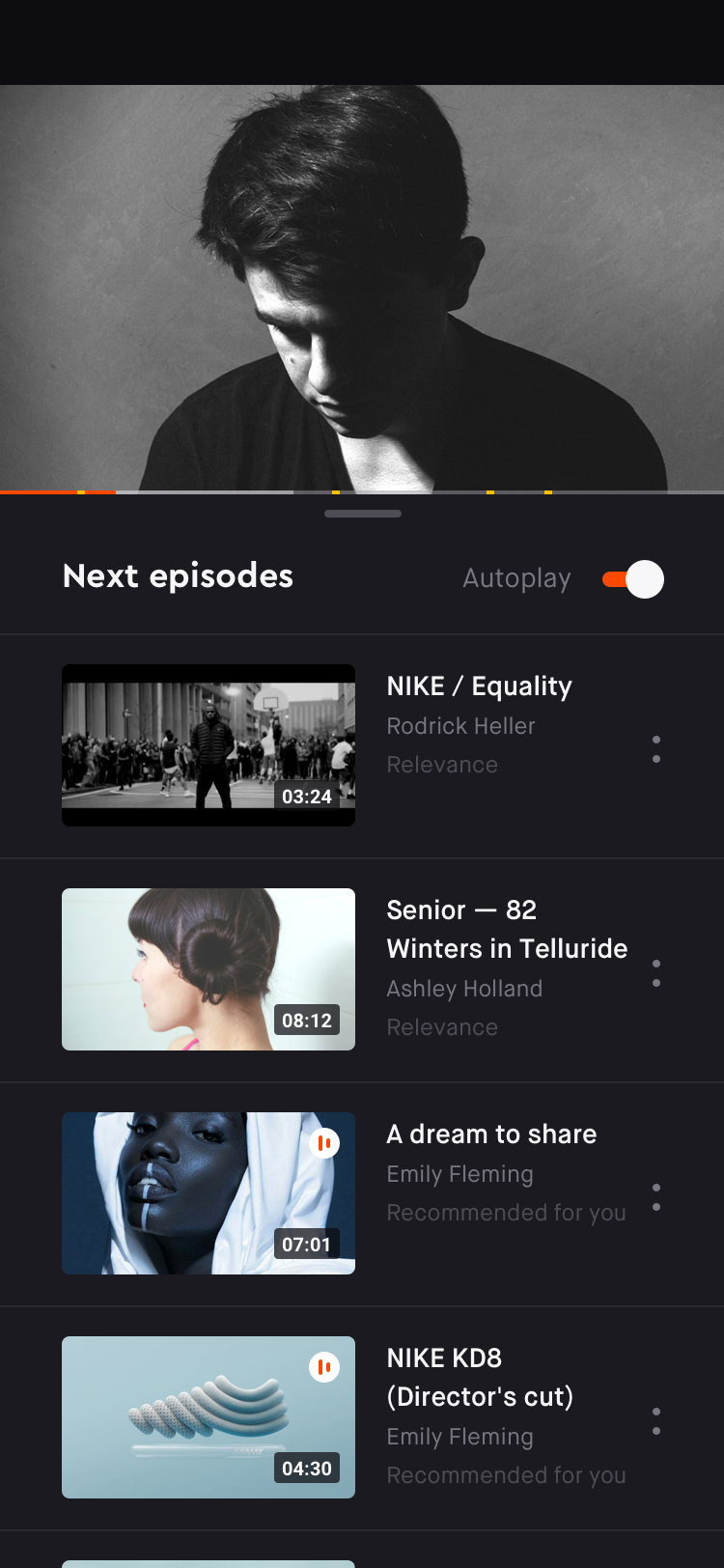A screenshot of a smartphone in a dim setting, predominantly featuring a black background. At the top, there's a black bar followed by a black and white image of a person with short brown hair, dressed in a black shirt, and illuminated by moody lighting while looking downward. The interface resembles a video player; a partially filled red progress bar at the bottom indicates ongoing playback, dotted with four yellow markers signaling ad placements. Below, the text reads "Next Episodes" and "Autoplay," with a toggled switch set to 'on'. 

Further down are thumbnails of four videos. 

1. A black and white thumbnail titled "Nike / Equality" featuring Roderick Heller with a label "Relevance" marked by two dots.
2. A person sporting a bun, titled "82 Winters in Telluride" with Ashley Holland, also marked as "Relevance."
3. An image of a person in a white hood with white makeup extending from their mouth to their chin, titled "The Dream to Share: Emily Fleming," labeled "Recommended for you."
4. A computer-generated image titled "Nike KD8 (Director's Cut)" by Emily Fleming, also labeled as "Recommended for you."

The interface suggests a content-sharing or streaming platform hinged on relevancy and personalized recommendations.